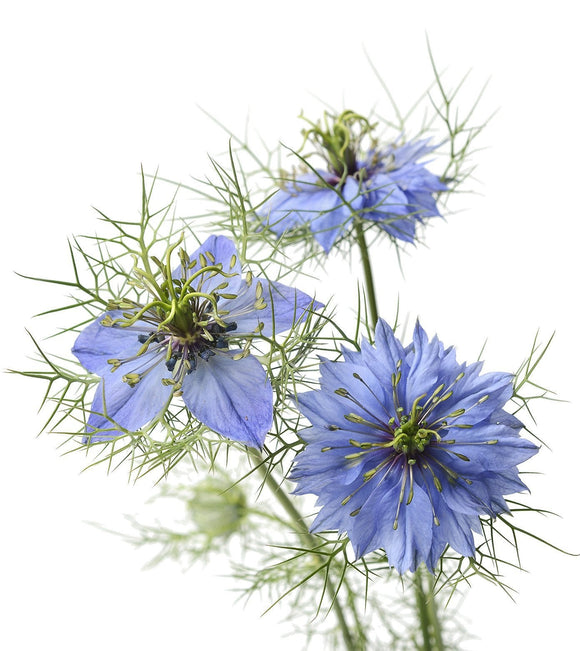In this picture, there are three flowers of the same species, each at different stages of blooming. The flower in the foreground, situated in the right lower corner, is densely filled with numerous purplish-blue petals that seem to be connected and layered, creating a rich, full appearance. In contrast, the flower to the middle left has only five petals, presenting a simpler structure. The flower in the background is slightly blurred but appears to have a moderate number of petals, falling somewhere between the two in the foreground. All three flowers are located on green stems adorned with thorny spikes that wrap around the petals. The tops of the flowers feature small, green sprigs where bees would typically pollinate, resembling tiny tentacles. Additionally, beneath the flowers, there are green, spiky appendages sticking out, adding to their intricate detail.